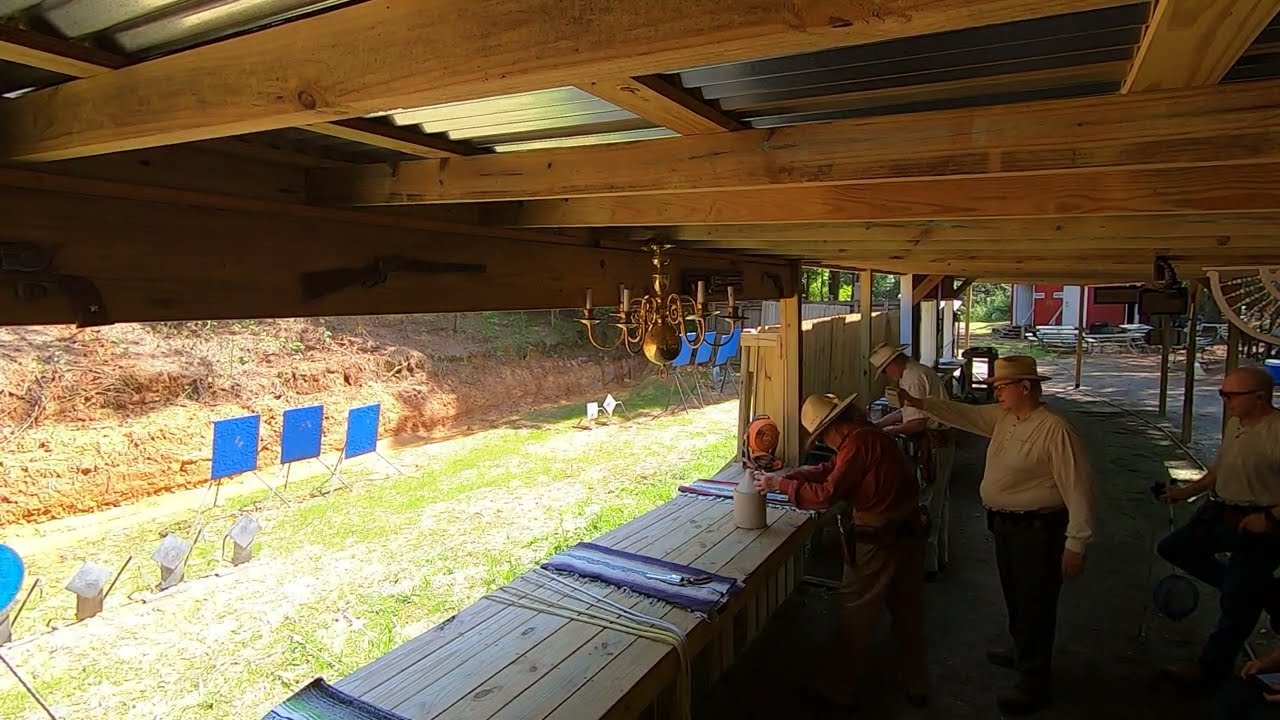Inside a rustic barn-like structure with a wooden and corrugated metal roof, four Caucasian men are gathered, engaged in various activities. Two men in large-brimmed cowboy hats are seated at a wooden table or bench, focusing on what appears to be gun preparation, with tools and possibly cloth or leather spread out nearby. Both are dressed in white shirts—one in long sleeves and the other in short sleeves—and black pants. 

A third man, also in a white shirt and donning a cowboy hat, stands with his right arm extended, pointing outside. He appears to be directing his attention toward a grassy outdoor area where square blue targets are set up, backed by hay bales. The floor near them is concrete, and a low wooden counter and wall partition off the area. 

The scene is lit by an unusual chandelier hanging from the ceiling, featuring candles. Additional lighting dangles from the wooden and metal beams above. In the background, the sight of a red building, likely another barn, can be observed, adding to the rustic ambiance of the setting. Multiple oil cans and additional easels with blue panels stand outside, further contributing to the impression that this might be a shooting range. A fourth man, leaning against the wooden wall, completes the group, creating a vivid tableau of a moment frozen in this industrious, rural environment.